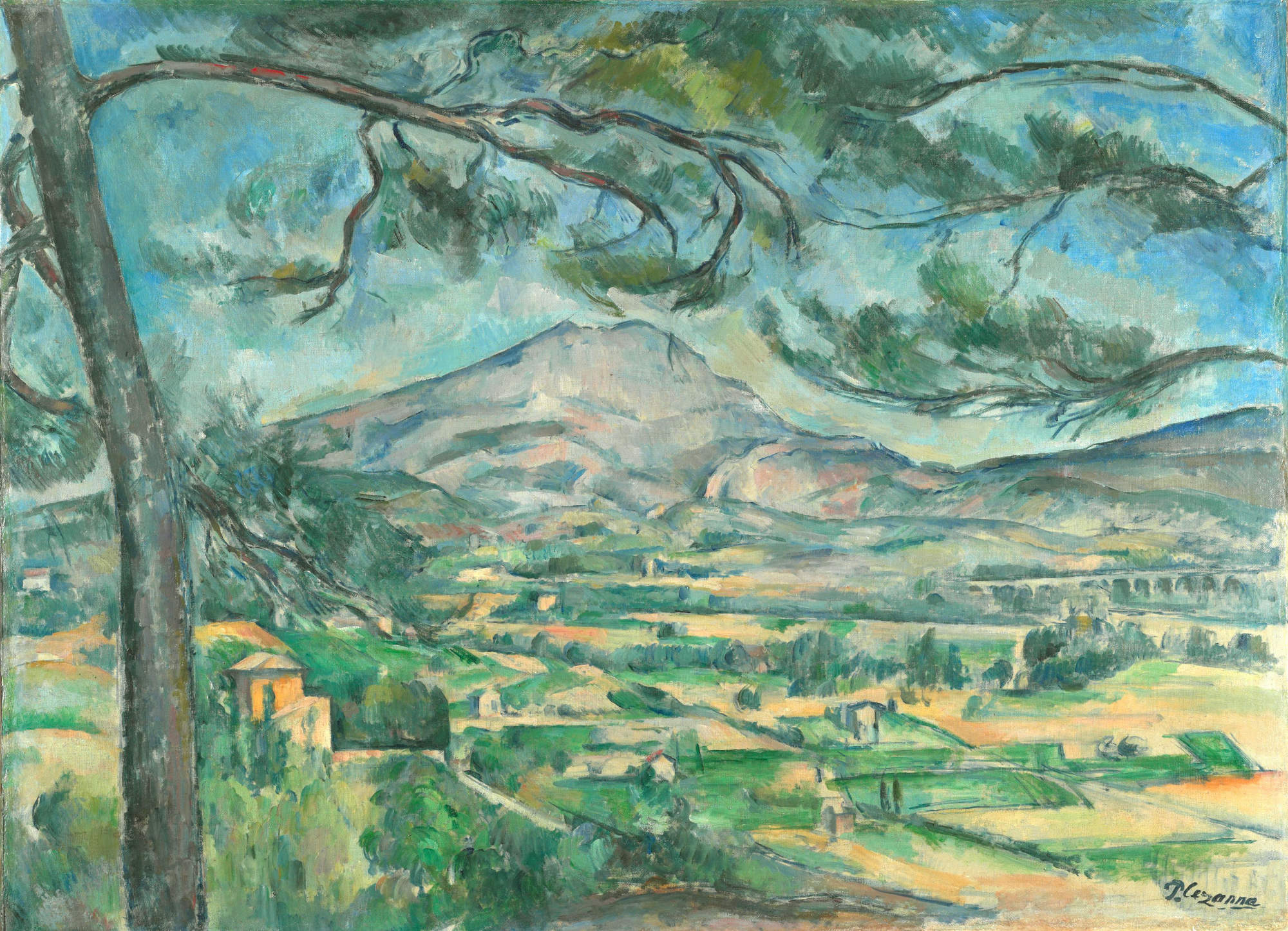This detailed painting showcases a vibrant rural mountainscape with a mix of natural and man-made elements. Hand-painted with noticeable big brush strokes, the image primarily displays a mountainous terrain with a predominantly green palette complemented by yellows and blues. In the foreground, on the left side, stands a thin pine tree with green spackled leaves and a grayish-brown trunk and branches. The tree's branches jut out on either side, with the ones on the left curving inward.

The midsection reveals a cluster of small, rectangular farmhouses scattered across flat fields of varied brown and green hues, suggestive of farmland. The artist captures the essence of a simple, rural community beneath a towering mountain, which exhibits shades of pink, green, and brown. The majestic mountain, central to the composition, contrasts with the bright blue sky above, dotted with white and gray clouds. An isolated bridge appears on the right, blending into the scene.

Adding an element of authenticity, the artist’s signature is found at the bottom right corner of the painting. The viewpoint suggests a slightly elevated perspective, giving the viewer a sense of looking down onto the serene, albeit abstract, rural landscape. Overall, this painting beautifully combines natural features with subtle human touches, creating a harmonious and peaceful rural vista.